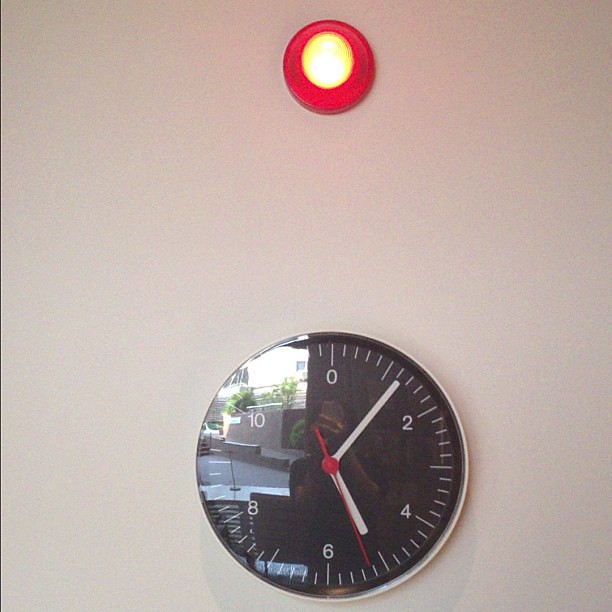A photograph captures a wall clock mounted on a gray-beige wall. The clock face is black, accentuated by white hour and minute hands, and a red second hand. The time displayed on the clock is 5:06. The glossy surface of the clock face reflects part of the outside world, revealing a parking lot with a distinct white car. Additionally, the reflection includes a faint image of the photographer. Positioned approximately a foot and a half above the clock is a light bulb, emitting a yellow glow and surrounded by a red base.